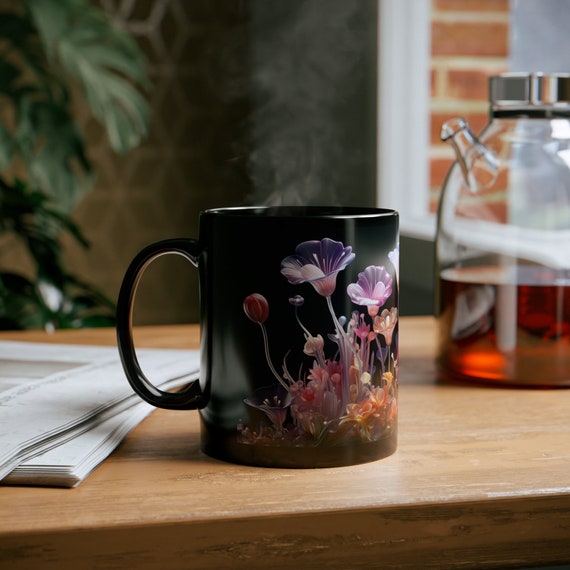This image captures a black coffee mug adorned with a beautiful floral print, prominently placed on a medium brown wooden counter. The mug, positioned slightly below center in the frame, features a handle on the left and a complex floral design, including delicate thin white stems, purple leaves, white leaves, small pink, yellow, orange, and green flowers, and an unopened pumpkin-like bud.

To the left of the mug sits a stack of off-white or light gray papers, possibly newspapers. On the right side of the mug, a bit blurred in the background, there's a clear glass pitcher with a silver lid, containing a light brown liquid that resembles apple juice or tea. Further in the background, slightly out of focus on the upper left, tall indoor palm leaves are visible. There is also a hint of an outdoor scene through a window on the right side, revealing red brickwork of a building outside. Steam can be seen gently rising from the coffee mug, adding a sense of warmth to the scene.